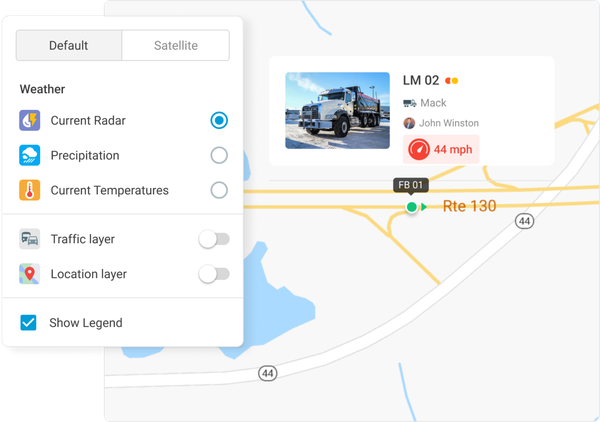The image depicts a detailed map from a website with various layers and settings. There is a pop-up overlay in the upper part of the screen, providing options such as "Divulge" and "Satellite," with the default set to "Weather." The pop-up indicates that the "Current Radar," "Precipitation," "Current Temperatures," and "Traffic Layer" options are available, with the "Show Legend" and "Current Radar" boxes ticked. The map beneath this overlay shows Route 130 and another intersecting road, with a highlighted truck traveling at 44 miles per hour on February 1st. This truck is identified as a Mac truck with the license plate "LM-02 John Wilson." The map itself features a color-coded legend: water bodies are blue, land is light tan, primary roads are mustard yellow or white, and various data points are marked in purple, yellow, blue, red, orange, green, teal, gray, white, and black hues.